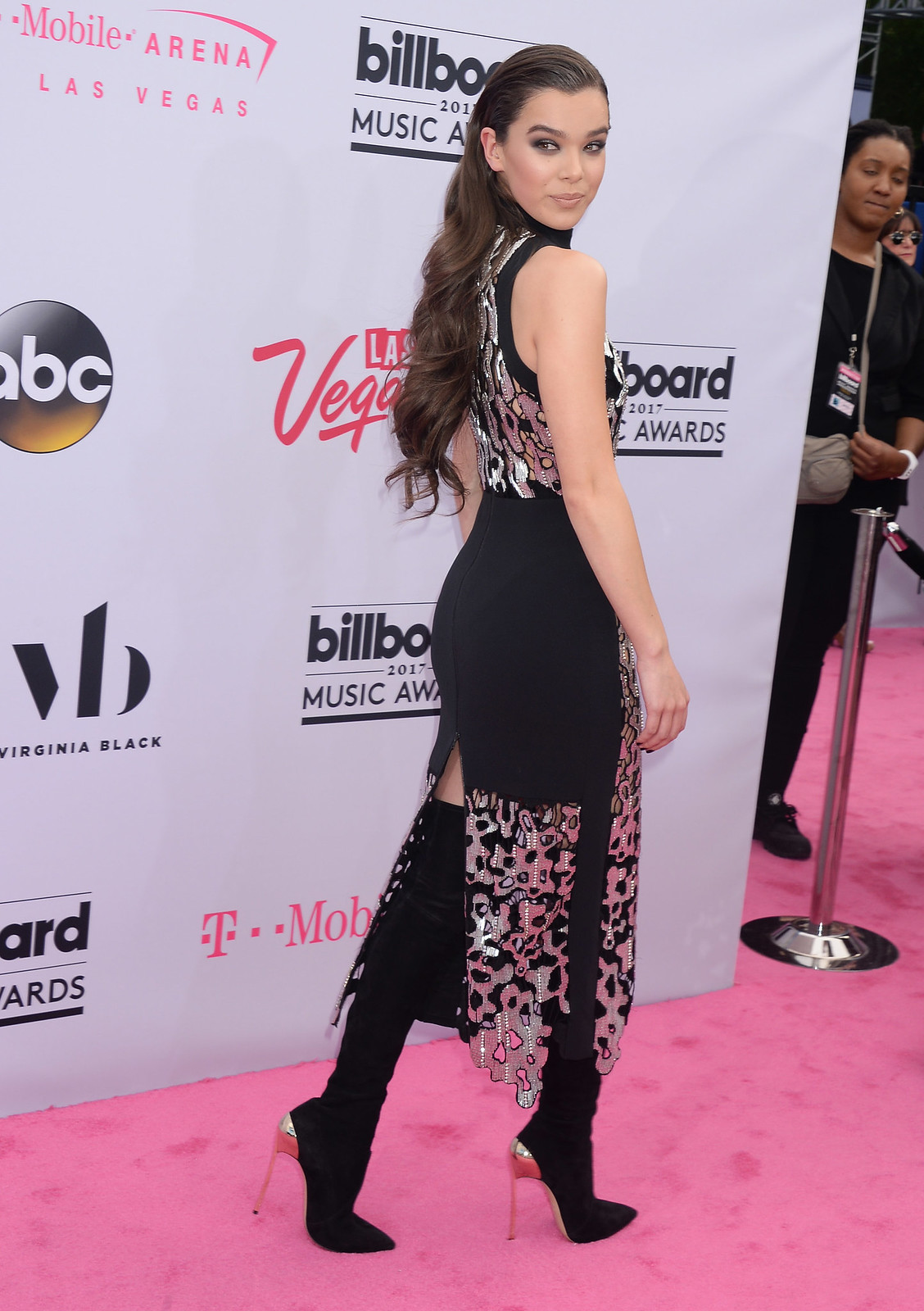The image captures a middle-aged woman, likely a model, actor, or singer, walking on a pink carpet at the 2017 Billboard Music Awards. She is exquisitely dressed in a black gown adorned with intricate silver patterns and sporting a stylish slit at the bottom. Complementing her outfit, she wears high heel shoes with silver tips. Her long, well-styled brown hair cascades down her back, and her smoky eye makeup accentuates her elegant look. She is looking back over her shoulder while walking, giving a captivating side-glance. This moment is set against a large white backdrop featuring logos such as ABC, T-Mobile, and various references to the Billboard Music Awards, Mobile Arena, and Las Vegas. In the distance, spectators can be seen behind a velvet rope. The polished setting and her sophisticated attire underscore the grandeur of the event.